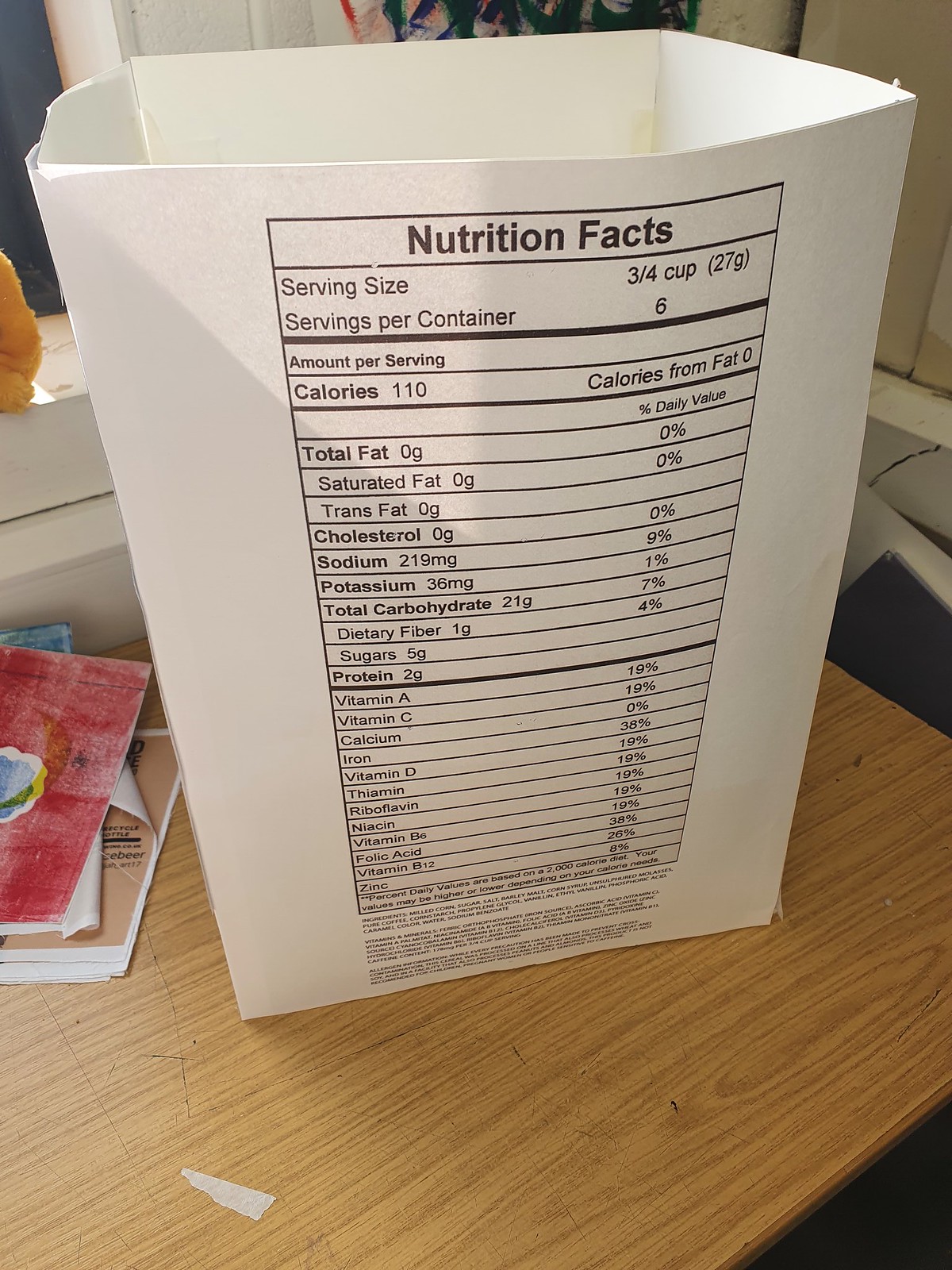This image features a clear photo of a white, rectangular cardboard package displaying a detailed Nutrition Facts label. The label specifies that the serving size is three-fourths of a cup, with six servings per container, and lists various nutrition details including calories, total fat, protein, cholesterol, sodium, potassium, total carbohydrates, sugars, and multiple vitamins along with calcium and iron. The box resembles a slightly larger version of a popcorn container, open at the top. It is placed on a rectangular, brown wooden table which appears to be resting on a blue and white surface. To the left of the box, there is a small stack of papers, which includes a few pamphlets or notebooks and what seems to be a piece of artwork. In the background, part of a white-painted windowsill is visible with an indistinguishable tan-colored object on it. The purpose of the box is not clear from the image.